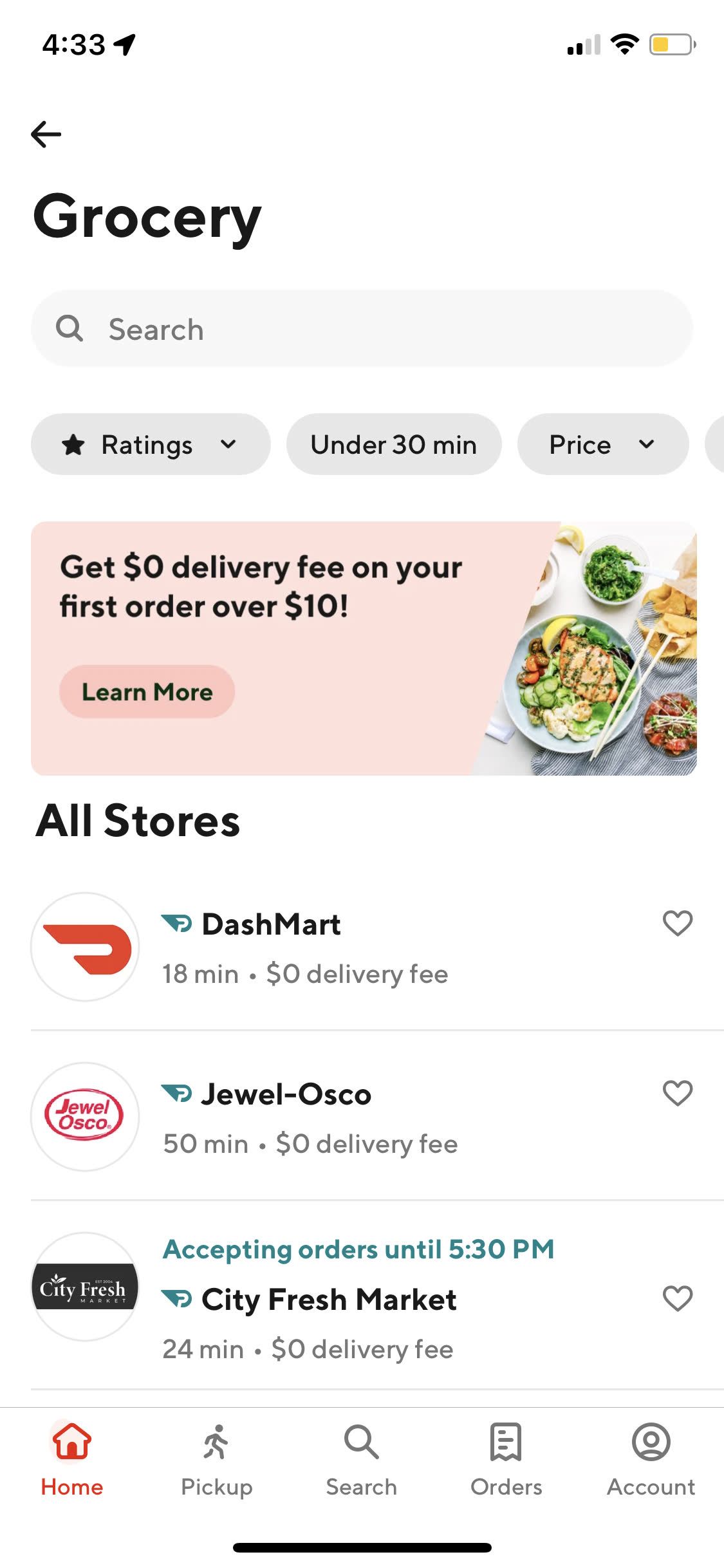The image is a detailed screenshot from the DoorDash app interface. At the very top of the screen, the time is displayed as 4:33, and to the right, there are icons for data signal, Wi-Fi connectivity, and a battery indicator showing less than half charge and colored yellow. Below this status bar, on the left side, there is a label that says "Grocery" followed by a search bar. Further down, a row of filter options is visible, showing "Ratings," "Under 30 Minutes," and "Price." 

A prominent pop-up window offers a promotion, stating, "Get $0 delivery fee on your first order over $10," with a "Learn More" button below it. Under this promotional banner, the app lists available stores: 

- "DashMart" with a delivery time of 18 minutes and a $0 delivery fee.
- "Jewel-Osco" with a delivery time of 50 minutes and a $0 delivery fee.

At the top of the list of stores, it mentions that orders are being accepted until 5:30 p.m. Below this is another store listing for "City Fresh Market," with a delivery time of 24 minutes and a $0 delivery fee.